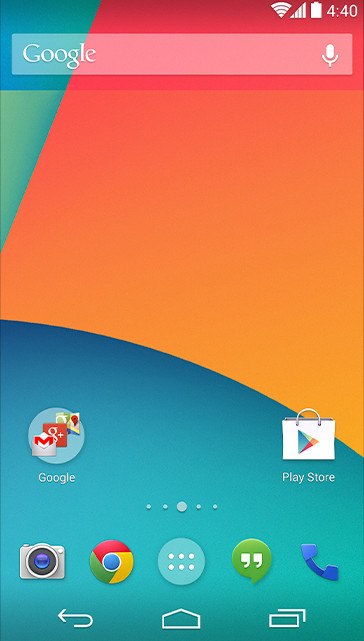The image shows a mobile phone display with several indicators and a vibrant, multicolored background. Starting from the top, the status bar includes a Wi-Fi icon, signal strength displaying four bars, a full battery icon, and the time reading 4:40.

The phone's wallpaper is visually striking with a combination of three main colors. At the bottom, there's a medium blue hue. Above that, from the upper-right corner, a red-to-light-orange ombre streak cuts across the screen diagonally, starting three-fourths of the way from the right and extending to the middle on the left side. On the right side, the ombre finishes three-fourths down the screen. In the top left corner, a small upside-down green triangle extends a couple of inches downward.

At the top of the display, a white text box contains the word "Google" followed by a microphone icon. The bottom of the screen features various app icons, including a Google Apps shortcut and a Play Store shopping bag. Below these, there is a row of individual app icons: a camera icon, a Chrome browser icon, a blue app with six buttons, a green app with two apostrophes, and a blue phone icon.

At the very bottom of the screen, there are navigation buttons in white: a back arrow, a home icon, and a recent apps overview represented by two overlapping rectangles.